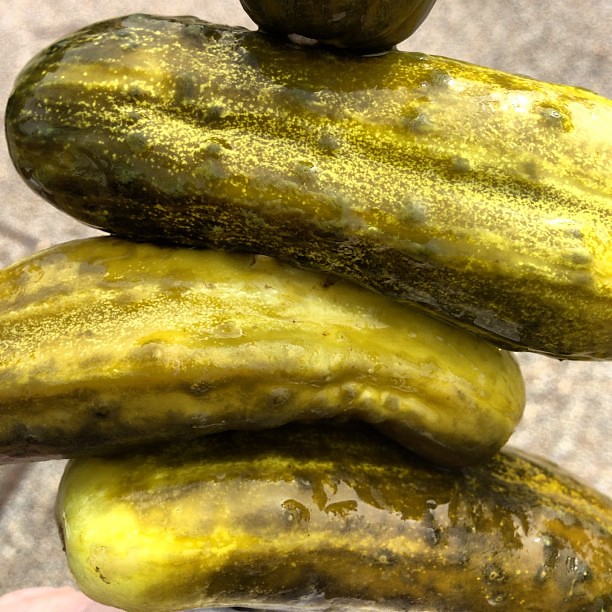The photograph, a vivid and textured color image, captures a close-up view of four sizable dill pickles, seemingly taken outdoors. These pickles, exhibiting various shades of green, are arranged lengthwise from left to right, stacking atop one another intricately. A small stick or spear pierces through them, possibly to keep them aligned. The top pickle is a dark green, flecked with pops of lighter, lime-green hues. Its textured surface is dotted with medium green bumps. The middle pickle, bathed in light, has a central region shimmering in lighter green tones, giving it a radiant appearance. The bottom pickle, glossy as if just plucked from pickling brine, features the same distinctive bumps. This lower pickle gleams brightly on the left side, adding to the image's captivating detail.